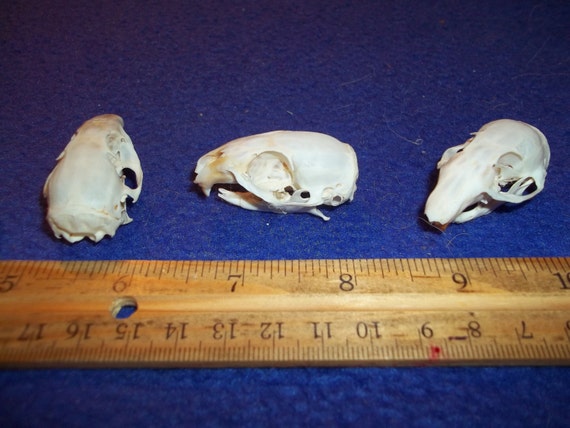This detailed photograph captures an indoor setting where the focal point is a close-up composition consisting of a wooden ruler and three small skulls, likely from rodents or small animals, displayed against a blue fabric background. The blue fabric, serving as a backdrop, is speckled with small white hairs.

The wooden ruler is positioned horizontally across the bottom of the image, showing measurements from just before the 5-inch mark to the 10-inch mark. The centimeter scale is also visible, inverted and stretching from approximately 17 centimeters on the left to nearly 6 centimeters on the right. A small hole is present between the 6-inch and 15-centimeter marks.

Above the ruler, the three white skulls are arranged at varying angles. The leftmost skull has its rear facing the camera, obscuring much of its structure. The center skull is oriented with the left side visible, its head turned to the left. The rightmost skull is positioned diagonally, with the nose pointing toward the bottom left of the image. Each skull features distinct eye sockets and pairs of sharp teeth, indicative of rodent or small animal species. The skulls measure roughly an inch to an inch and a half in length and about three-quarters of an inch in width, emphasizing their diminutive size against the ruler for scale.